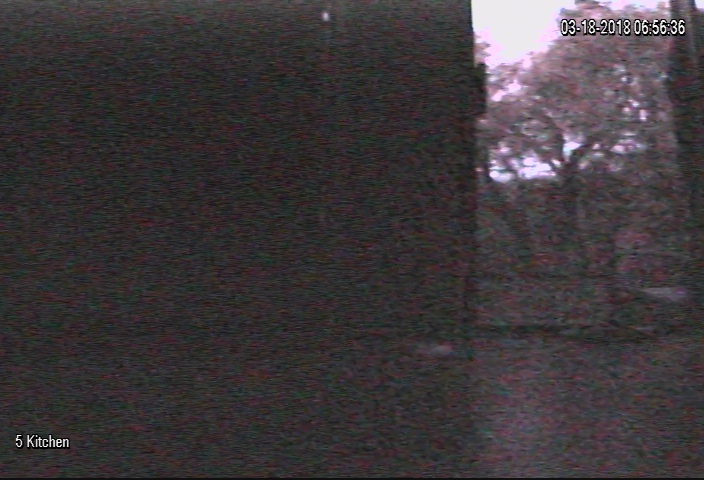This grainy, blurry image appears to be captured by a security camera aimed either within or towards a kitchen area, as indicated by the label '5 Kitchen' in white lettering at the bottom left corner. The scene is mostly obscured by a large, dark square object that spans approximately 70% of the image, stretching from the left edge to the center. Despite the poor quality with flecks of pink and gray scattered across the dark area, some details are visible on the right side: a tree adorned with pink petals, likely set against a backdrop of silhouetted hills. The top right corner displays a timestamp reading '03-18-2018 06:56:36,' suggesting the photo was taken early in the morning.